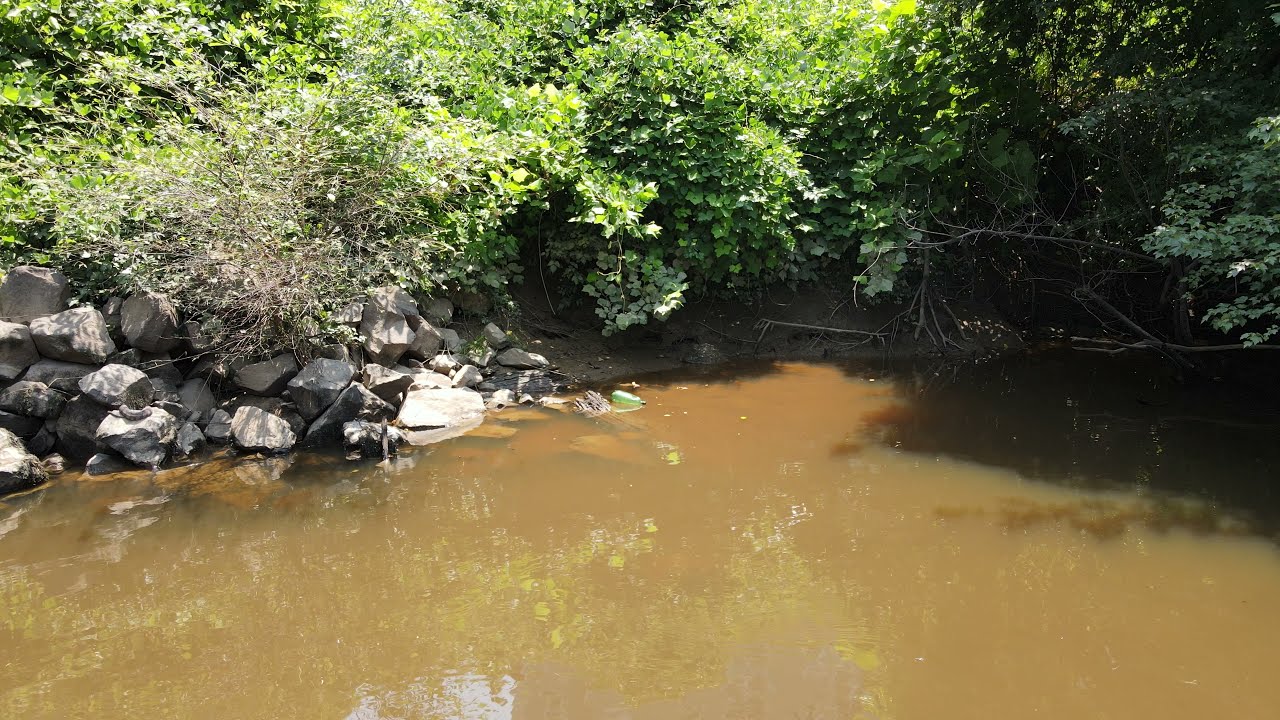This photograph, taken in landscape orientation at eye level, visually captures a muddy brown creek or river flowing from the mid-right center toward the foreground, where the water widens, forming a foreground dominated by murky, yellowish-brown water. On the left side, a rocky ridge rises from the water, covered with green shrubs and vegetation that are partially cast in shadow. To the right, a dense line of tall trees extends from the mid-horizontal right area to the upper right corner, casting shadows over the water. These trees appear more distant and heavily packed compared to the nearby vegetation. The background is filled with a thick layer of dense green trees and foliage, narrowing as it recedes. Sunlight illuminates the upper left area, creating a vivid contrast with the shadowy left bank of the creek. In the water, amidst the mud and dirt, a plastic bottle can be seen floating, while twigs and branches are scattered near the rocky sections of the banks. The overall scene suggests a forest or wooded area that is perhaps part of a farm or natural reserve, lit by daytime sunlight emphasizing the vivid greenery juxtaposed against the dirty, copper-colored water below.